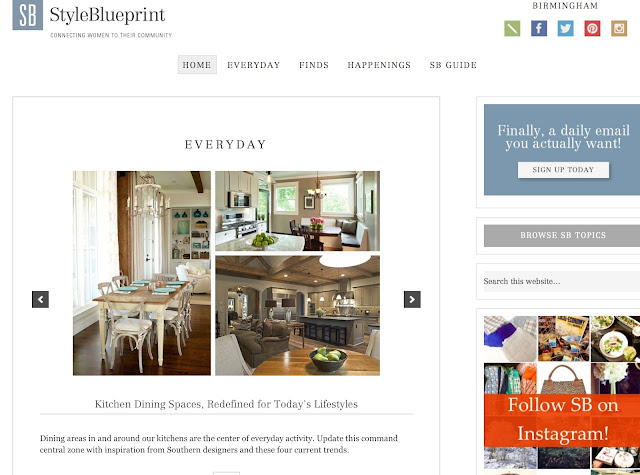This image showcases a web page from StyleBlueprint, a platform connecting women to their community, as indicated by the "SB StyleBlueprint" logo in the upper left corner. In the top right corner, the word "Birmingham" is displayed alongside several social media icons. The icons include a pencil inside a square, the Facebook logo, the Twitter logo, the Pinterest logo, and a brown square likely representing a camera icon. Below this header, the navigation bar highlights "Home," along with options such as "Every Day," "Finds," "Happenings," and "SB Guide."

On the left side of the page, there are three images showcasing different interior views. The first image features a dining area with a stylish dining table surrounded by multiple chairs. The second image provides a glimpse of a modern kitchen with visible appliances and an additional eating space. The third image captures a view from the living area looking into the kitchen, highlighting an island and a table in the foreground.

On the right side of the page, a promotional section invites users to sign up for daily emails with a compelling tagline: "Finally, a daily email you actually want. Sign up today." Additionally, there are prompts encouraging users to explore "SB Topics," search the website, and follow StyleBlueprint on Instagram. The content underlines the theme of redefining kitchen and dining spaces for contemporary lifestyles.